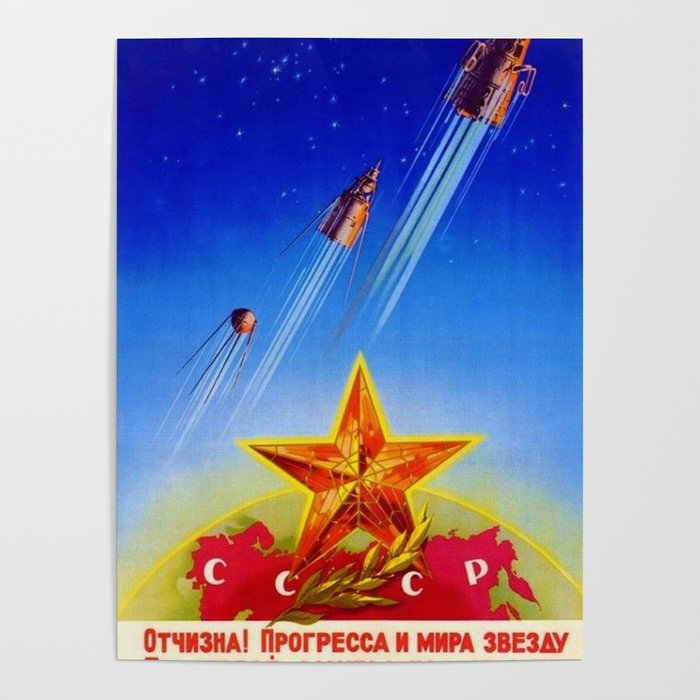This vintage poster features a central illustration set against a white background, bordered in gray. At the heart of the image is a large, stylized five-pointed star depicted in shades of orange, red, and gold, emitting a yellow glow. Positioned below the star, the text "CCCP" is prominently displayed in white letters on a red background, referencing the Soviet Union (USSR). Beneath this, there's a tan strip with additional text in Cyrillic, but its exact content is difficult to discern.

The upper section of the poster transitions into a gradient sky, shifting from light blue at the bottom to a much darker blue at the top, symbolizing the expanse of space. Dominating this area are three chrome-colored rockets blasting upwards, leaving trails as they ascend. Surrounding these rockets, various satellites can be seen, scattered among stars in the dark blue expanse, emphasizing the theme of space exploration.

Overall, the poster showcases a bold, patriotic display of Soviet space achievements, with a focus on the glory and technological prowess of the era.